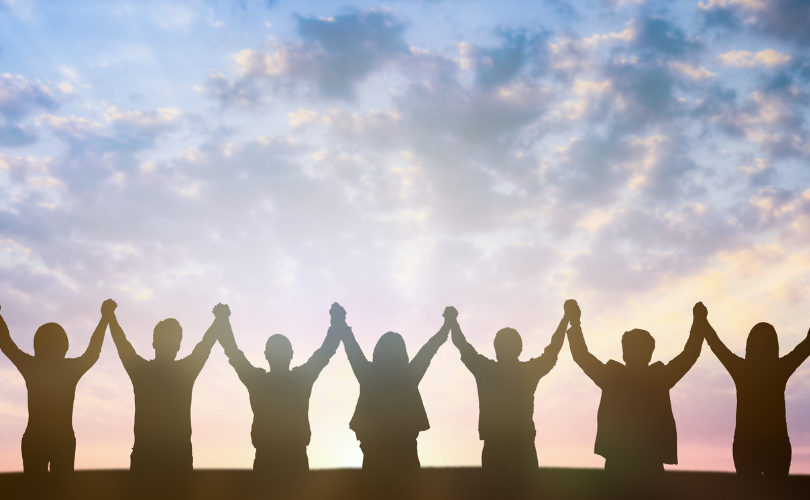In this evocative photograph, seven individuals, silhouetted against a pastel sky, stand in a line holding hands with their arms raised in a Y-shape, symbolizing victory. The image, taken from behind, captures only the darkened outlines of their figures, emphasizing their unity and collective gesture. The sky above them is a mesmerizing blend of colors, with pink and light yellow hues at the horizon gradually transitioning into shades of purple and blue, adorned with fluffy clouds. The sun, either rising or setting, casts an ethereal light that frames the scene, highlighting the tranquil and inspiring moment amidst the serene pastel-colored sky.